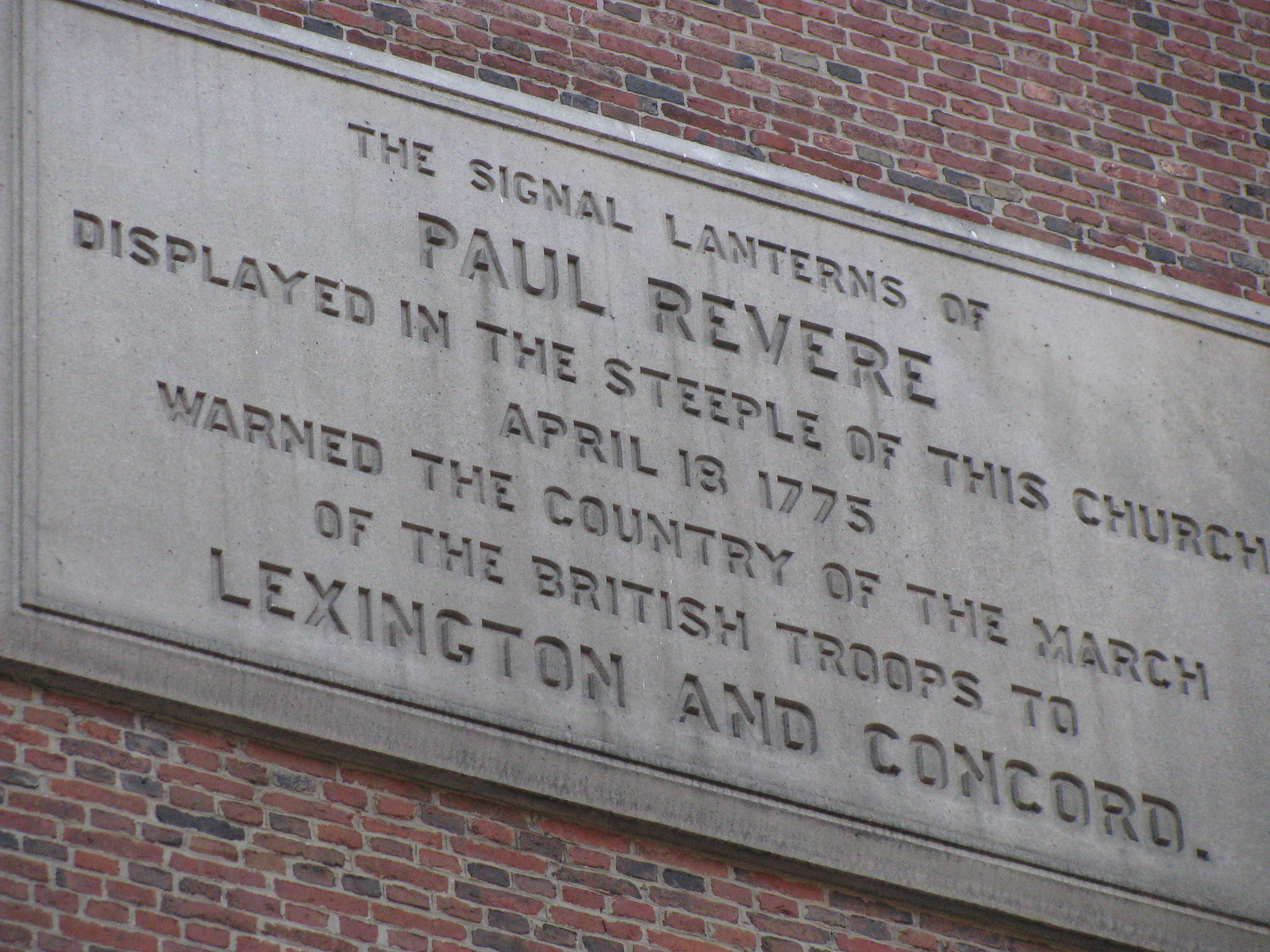The image captures a close-up of a historical plaque affixed to a red brick wall, the bricks varying in shades from red to gray. The plaque itself is large and made of gray stone, prominently contrasting against the brick background. The stone features a chiseled-in border that frames the six lines of text, which are carved into the stone in the same color but have become blackened around the edges due to age. The text reads: "The signal lanterns of Paul Revere displayed in the steeple of this church, April 18th, 1775, warned the country of the march of the British troops to Lexington and Concord." The words "Paul Revere" and "Lexington and Concord" are larger than the rest, highlighting their significance. The plaque is tilted from the upper left to the bottom right, creating a dynamic angle in the photograph.